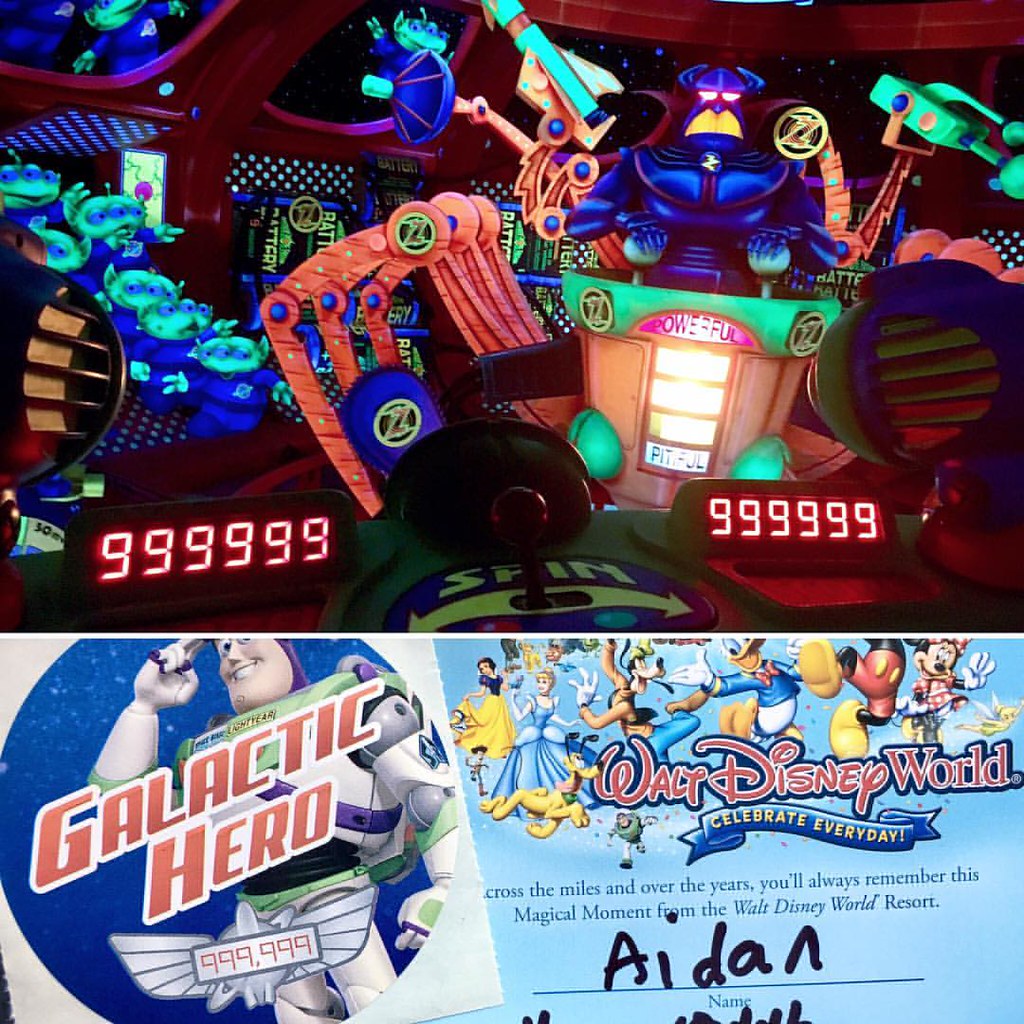This image is a card featuring two detailed video game scenes. The top scene showcases a blue, muscular animated figure with a stylized dog head and ears, underlined by a sign reading "Powerful Pit Bull." This figure stands atop what resembles a pinball machine, flanked by six robotic legs with mechanical joints. To each side of the figure are digital monitors displaying a sequence of six nines ("999999"). In the backdrop, a row of digital screens display various graphics, including a rocket against a space-themed background. 

The bottom half of the card is split into two sections. The left side features Captain Buzz Lightyear from Toy Story with the label "Galactic Hero." On the right, there is a montage of Disney characters with the text "Walt Disney World" above. Below, it reads, "Across the miles and over the years you'll always remember this magical moment from the Walt Disney World Resort," signed by Aiden in what appears to be a child's handwriting.